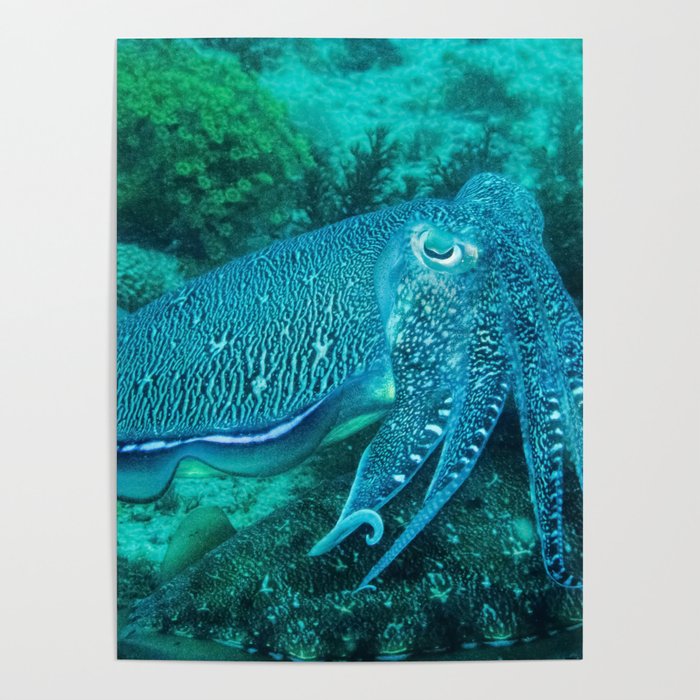In this large square image with a solid light gray background, a vertical rectangular underwater photograph forms the central focus. The photograph features a mysterious sea creature that may be an octopus, squid, or jellyfish, exhibiting vivid colors and intriguing anatomy. The animal’s body, primarily teal green with white edges, transitions to blue shades highlighted by lighter blue streaks. Its eyes are prominently positioned on top of its head; they are translucent with black and white layers, suggesting a jelly-like coating over them. Multiple arm-like flaps, resembling octopus arms, protrude from its face, with four clearly visible on the right side before the image cuts off.

The underwater scene is bathed in a greenish hue, lending a sense of depth and immersion. The background is somewhat grainy and detailed, featuring a variety of plants on the ocean floor in diverse shades of green—bright green, light green, and darker green. Yellow, flower-like structures and a gray to tan sandy bottom add to the seascape’s richness. Also present are gray and white rocks on the bottom right and other colorful reefs, completing the exotic marine environment.